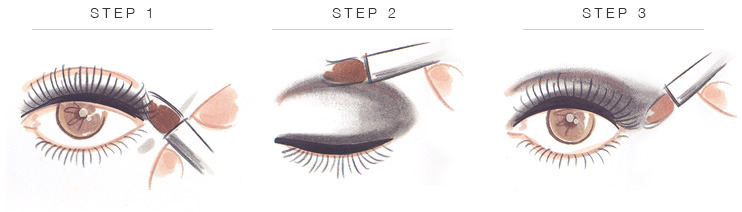This rectangular, landscape-oriented image provides a detailed step-by-step guide on applying eyeliner, presented through three separate, cartoonish illustrations of a brown eye. Each step is distinctly labeled at the top in all caps as Step 1, Step 2, and Step 3, each underlined with a light gray line.

- **Step 1:** Shows the eye open, with a thin brush being positioned above the eyelashes, ready to apply the eyeliner.
- **Step 2:** Depicts the same eye now closed, with the brush being pulled from left to right across the eyelid, marking the application process.
- **Step 3:** Displays the eye open again, showcasing the completed eyeliner application above the eye.

The entire guide employs a minimalist color palette of brown, black, white, and gray, and prominently features the brown eye and the brush with a brown applicator, handled by fingertips approaching from the right side of each image. The overall style resembles a colored pencil drawing, focusing on the essential actions in each step to effectively illustrate the eyeliner application process.